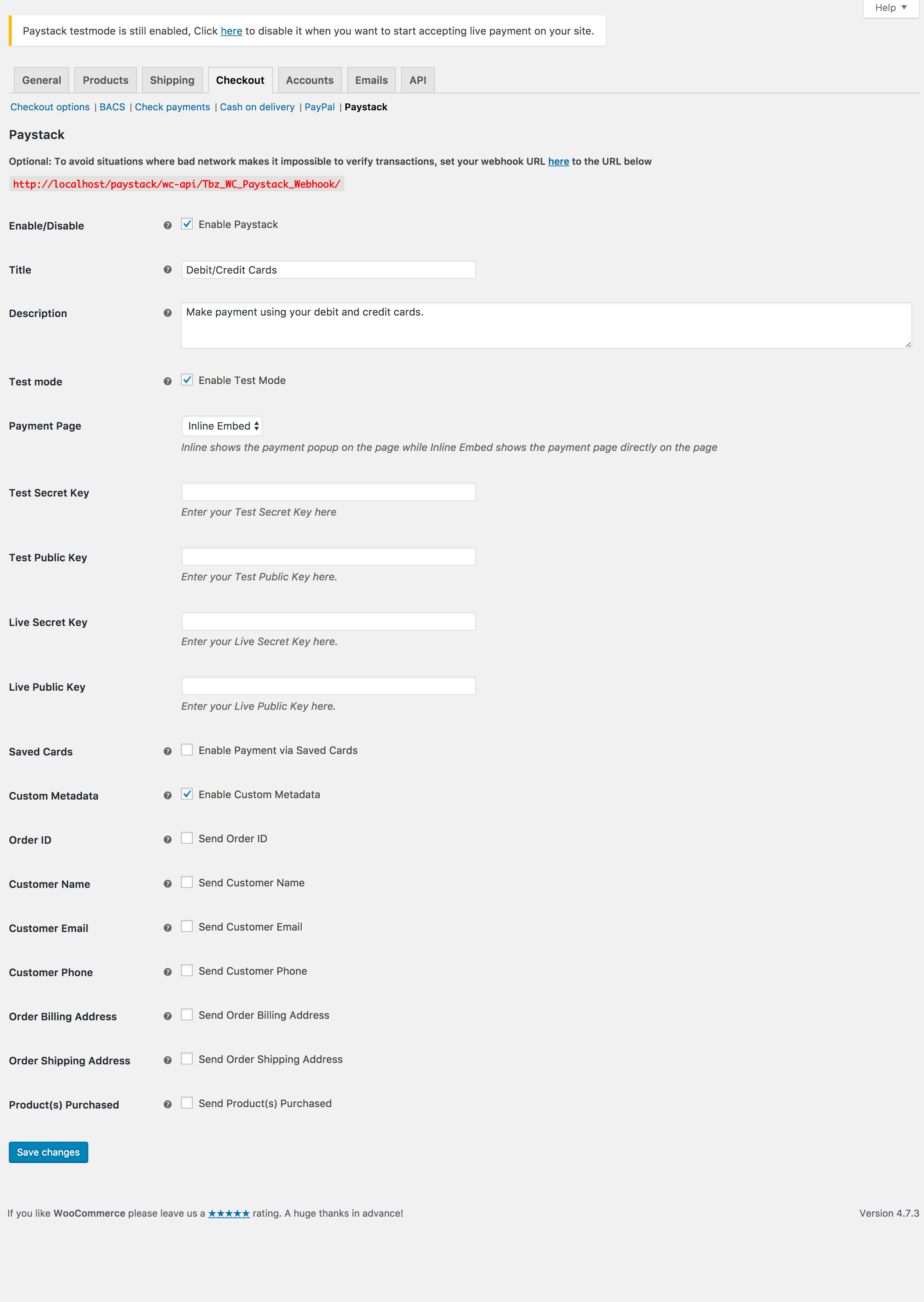A screenshot of a website's backend interface for setting up payment options is shown. The screen is titled "Payment Screen Setup" and presents various fields and options for configuring payment methods. At the top, a notification indicates that "Payback Test Mode is still enabled" and advises users to click to disable it when ready to start accepting live payments. The interface lists various payment options, including "Paystack," with individual configurable attributes such as "Enable," "Disable," "Title," "Debit Cards," and "Description." Approximately 20 fields are displayed, all with a gray background and white input areas. At the bottom left corner, a "Save Changes" button is visible, allowing users to save their configuration adjustments. The top of the screen features a set of tabs labeled "General," "Product," "Shipping," "Checkout," "Accounts," "Emails," and "API" in black text. The overall setup highlights the detailed customization options available for managing payment settings on the website.